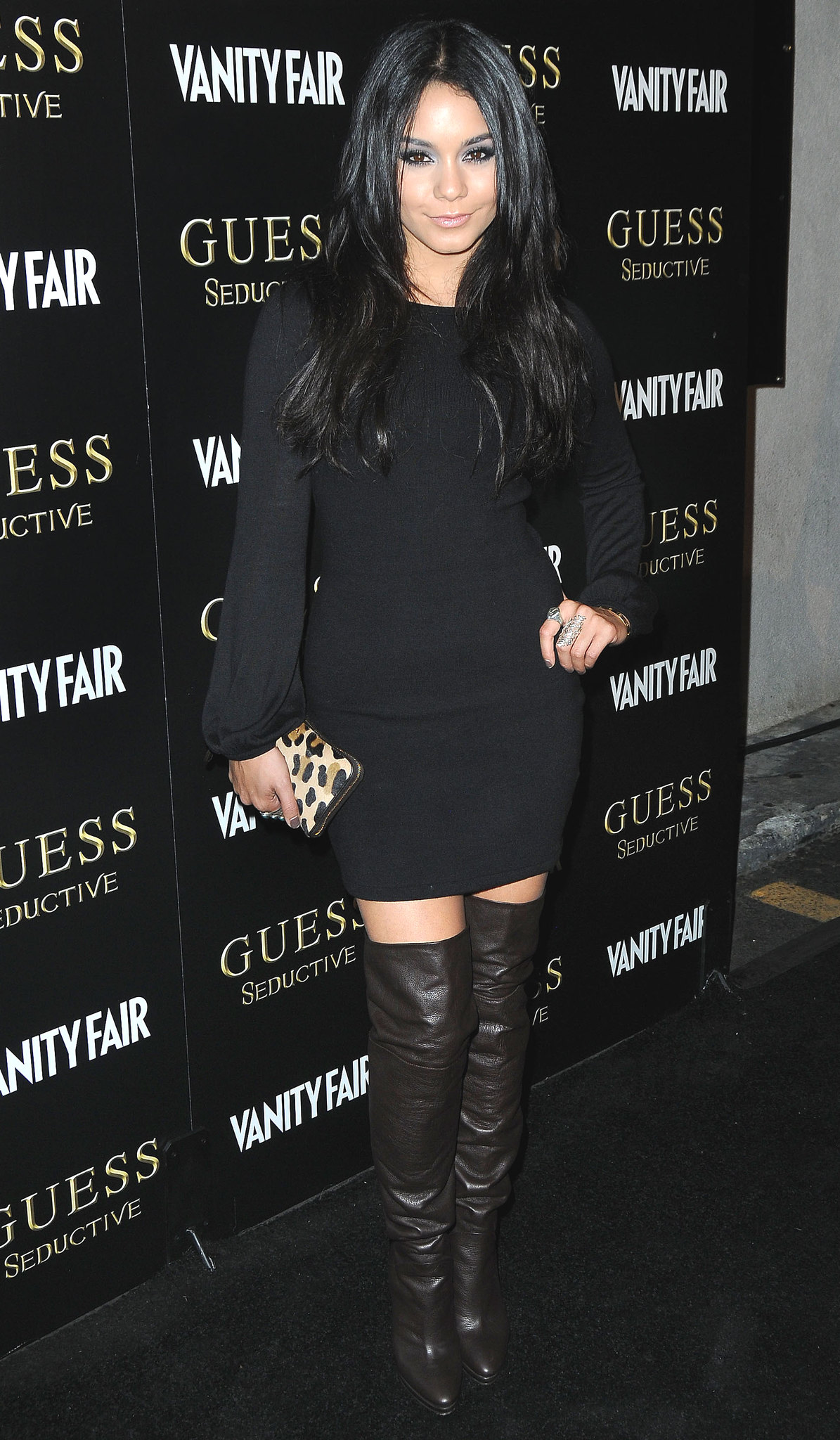In this image, Vanessa Hudgens is standing confidently at the center, posing for photographers against a black-themed backdrop. Her outfit is chic and fashionable, featuring a short black sweater dress paired with thigh-high black boots. Vanessa's dark, shiny hair cascades to her shoulders, complementing her makeup, which includes eye shadow and lipstick. She has one hand placed on her hip, displaying rings on her fingers, while the other hand holds a leopard-print purse, adding a touch of pattern and color to her ensemble.

The background features a three-panel wall adorned with alternating advertisements for "Vanity Fair" and "Guess Seductive," both written in white against the black partitions. The repeating text runs from the top to the bottom of the wall, creating a striking and cohesive visual effect. The setting is an indoor event, possibly a modeling or award show, as suggested by Vanessa's poised stance and the professional backdrop. The carpet beneath her mirrors the black tones of her attire and the wall behind her, creating a unified and stylish scene. Vanessa looks directly at the camera, offering a subtle smile, making it a seemingly formal yet engaging photograph.